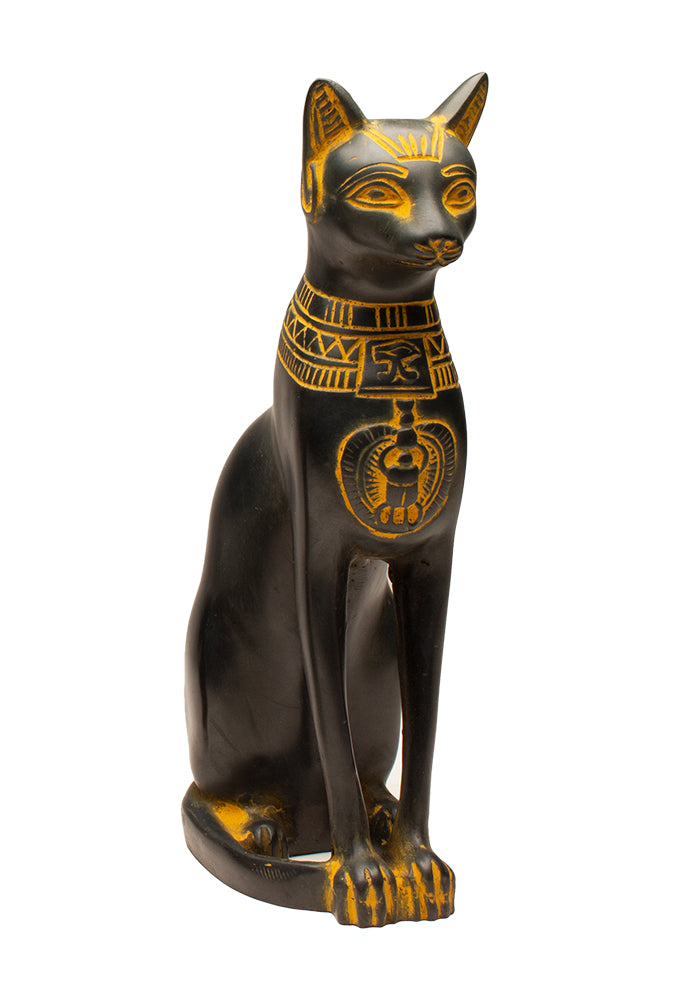This highly detailed statue represents a sleek, tall cat, reminiscent of ancient Egyptian art. The cat is meticulously carved from a dark, likely wooden material, boasting a shiny black finish. It sits elegantly on its haunches, with its front legs straight and ears perked up, exuding a majestic aura.

Gold accents embellish various features: the eyes, eyebrows, and the interior of the ears all have intricate gold inlays, while the nostrils and even the toes are highlighted with gold detailing. The cat's forehead features a golden crown-like design that further enhances its regal appearance.

Around its neck, the cat wears a grand, ornate collar or necklace designed with layered patterns, including zigzagging triangular motifs and straight lines, adding to its opulence. This necklace is approximately three inches thick and includes a circular medallion, about three to three and a half inches in diameter, that dangles prominently. The medallion features a dung beetle, or scarab, a symbol of renewal and revered in Egyptian culture, presented in black with gold accents.

Overall, this statue captures the essence of ancient Egyptian reverence through its detailed craftsmanship and symbolic adornments.